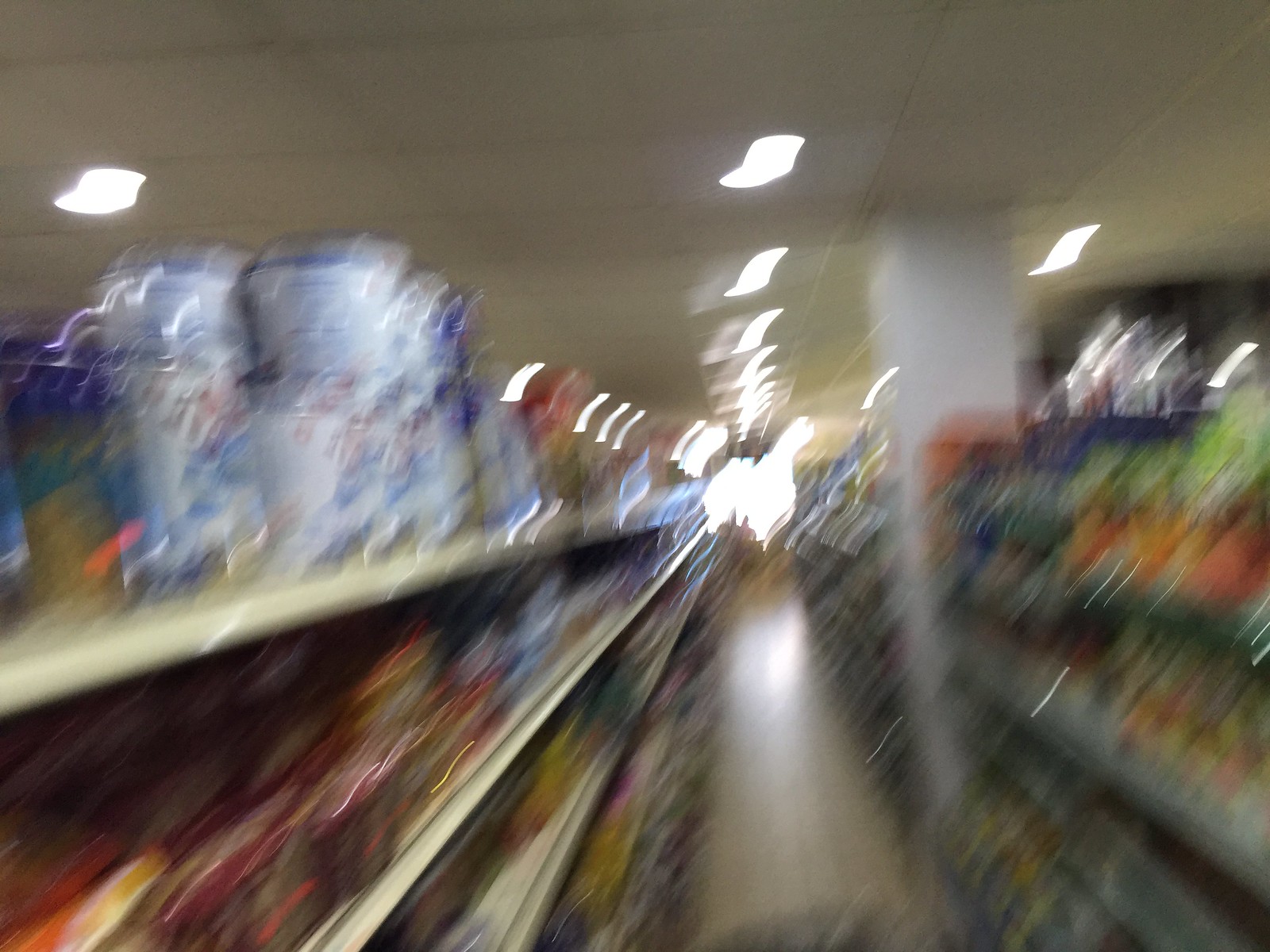This image portrays an extremely blurred view of a grocery or retail store aisle. The perspective is from the center of the aisle, looking down towards the far end. On either side of the frame, there are shelves stocked with various products, although the blur makes it difficult to discern what exactly is on them. In the foreground at the top shelf, there appears to be plastic packaging that possibly contains bottles of water. At the end of the aisle, a bright white light illuminates the area, and there seems to be a silhouette of two people standing, gazing back towards the observer. The ceiling lights are heavily blurred, and a support post is visible midway down the aisle. Overall, the image captures a retail setting in a highly obscured manner, making detailed identification challenging.